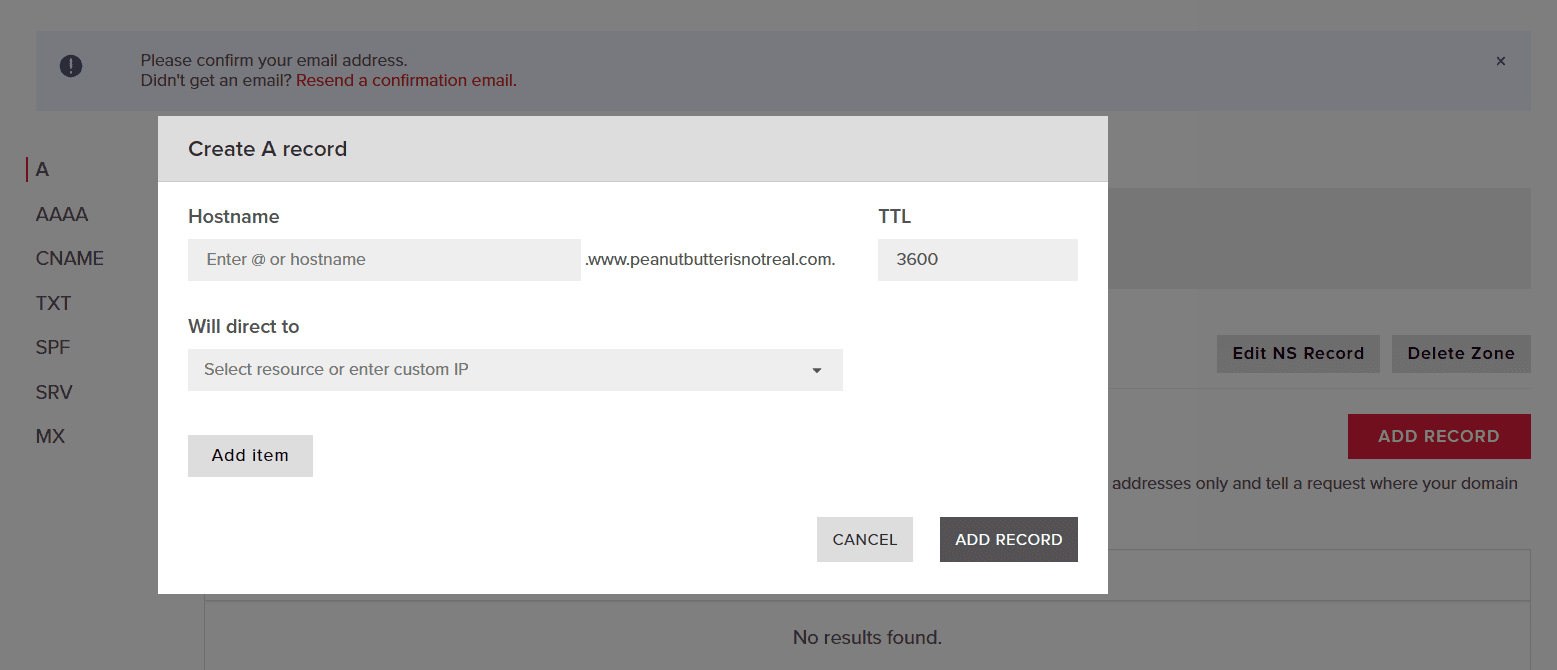The image shows a partially obscured web page covered by a thin gray overlay, featuring a prominent white box in the center of the screen. In the background, an information icon and a notification prompt, "Please confirm your email address. If you didn't get an email, resend a confirmation email," are visible. The left sidebar of the page contains a vertical list of tabs labeled: "Application A" (highlighted with a red bar), followed by "AAAA", "CNAME", "TXT", "SPF", "SRV", and "MX" in uppercase letters. 

To the right of these tabs, there are options for "Edit NS Record" and "Delete Zone," along with a red "Add Record" button. Below these elements, the section becomes less readable due to the overlay, but it concludes with a message saying "No results found."

The foreground box has a gray border and white background, titled "Create a Record." Inside, there are fields labeled "Host Name" with an input box for "@" or another hostname. Next to this field, it reads "www.peanutbutterisnotreal.com" followed by "TTL" and a box containing the number "3600." Below this is a dropdown menu labeled "Will direct to," which allows the selection of a resource or entry of a custom IP. At the bottom, there are buttons labeled "Add an Item," "Cancel," and "Add Record."